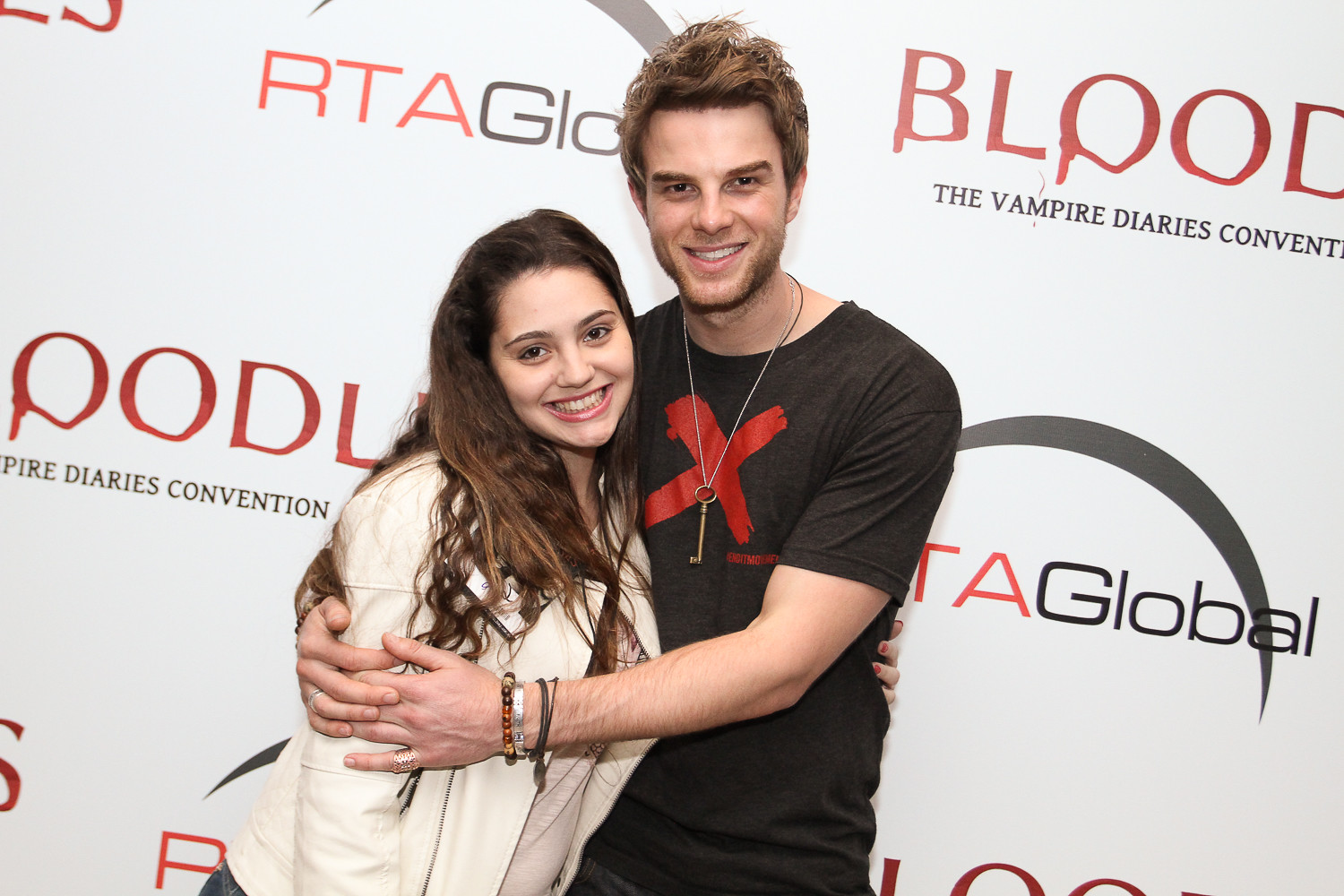This detailed photograph captures a moment at what appears to be a convention related to "The Vampire Diaries," possibly titled "Blood Something." The backdrop prominently features logos and text indicating RTA Global as a sponsor. In front of this backdrop, there is a man on the right side and a woman on the left, both of whom are smiling and clearly posing for the picture. 

The man is wearing a black t-shirt with a distinct red 'X' across it and has a necklace adorned with an old-style skeleton key. He has brown hair and both of his arms are wrapped around the woman. The woman has long, darker brown hair that partly obscures her name tag. She is dressed in a white jacket over a gray or white shirt and has her left arm affectionately placed around the man's mid-arm area. Both individuals are Caucasian and are engaging with the camera, suggesting a friendly and warm encounter, potentially between a celebrity and a fan at this well-organized event.